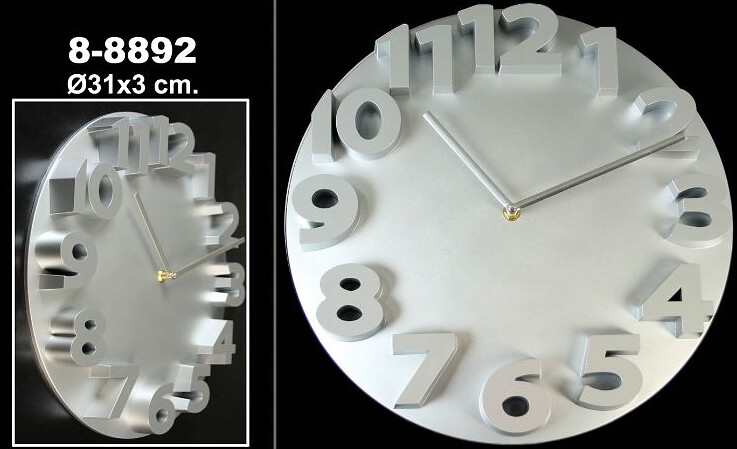This image showcases a clock viewed from two distinct angles. On the right side, there is a larger, square, straight-on view of the clock face, while on the left side, a rectangular perspective reveals the clock at a slight angle, emphasizing the raised, sculptural relief of the numbers. The clock's face, hands, and numbers are all rendered in white with a silvery metallic sheen, and the metal that holds the hands in the center is gold. Above the side view, white text reads "8-8 8 9 2", and below it, "0 3 1 x 3 centimeters." The large, elevated numbers are clearly seen pointing to an approximate time of 11:10.